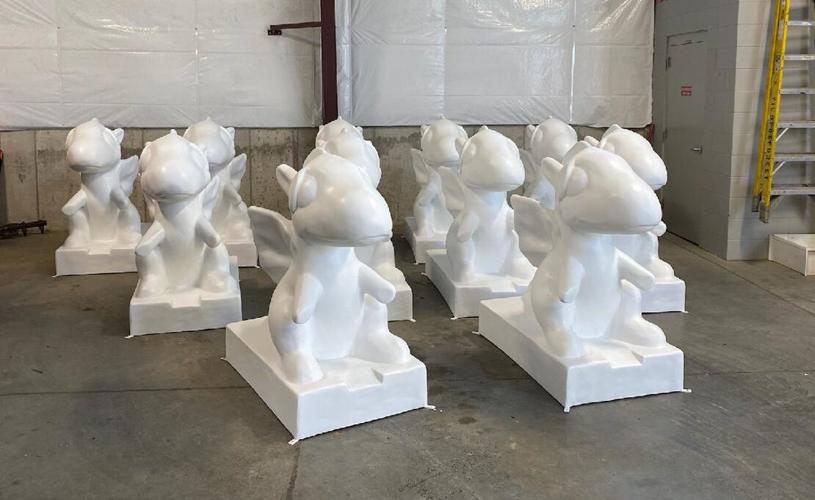The scene is set in a warehouse with concrete floors and a gray, cement-like ambiance. In the center, there are ten to twelve identical, unfinished statues lined up in a pyramid shape—two in the front, four in the next row, and four to six at the back. These statues represent a small, cute, and friendly-looking dragon, characterized by its round, bulbous head, small wings, short and stubby arms, and rabbit-like legs. The creature has a long snout, small angled-back ears, and appears stout with a notable small horn or spine atop its head. The statues are pure white, suggesting they are unpainted molds, possibly intended for promotional purposes. A yellow ladder is visible at the back right of the warehouse, adding to the industrial setting.